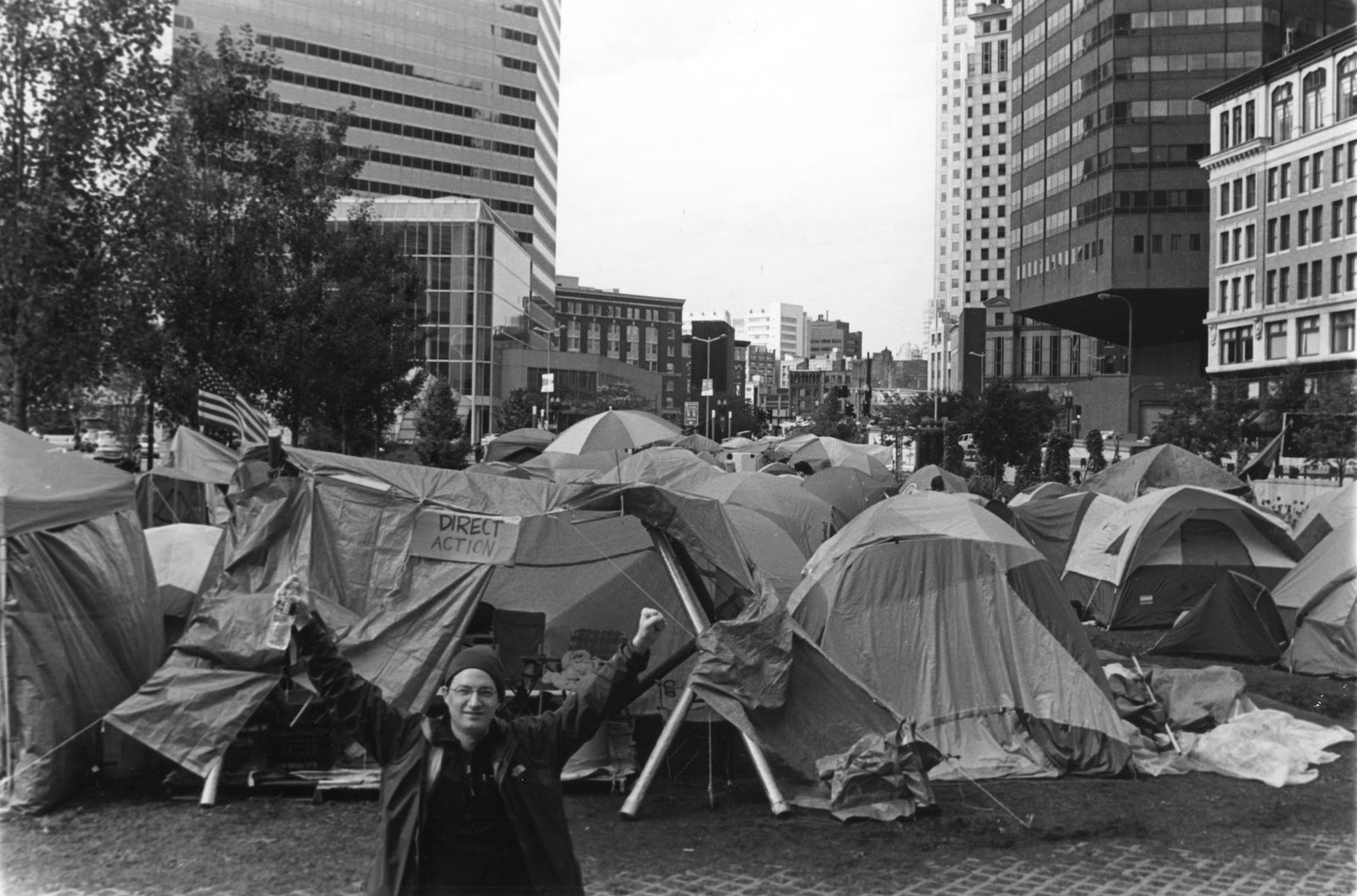This black-and-white photograph captures a protest campsite set in a bustling downtown area. In the foreground, a man stands prominently, wearing a toboggan and glasses, sporting dark clothing. He raises both arms—one holding a water bottle, the other a clenched fist—appearing to advocate passionately for a cause. Behind him, a myriad of tents line the street, suggesting a large gathering possibly involving around 30-50 camps. Among these tents, a conspicuous sign reads "Direct Action," emphasizing the protest's assertive nature. Nearby, blankets and other personal items are scattered, creating a lived-in atmosphere. The backdrop features towering skyscrapers, hinting at the urban setting, and trees visible to the left. An American flag waves in the vicinity of the trees, adding a poignant touch to the scene of civil demonstration.